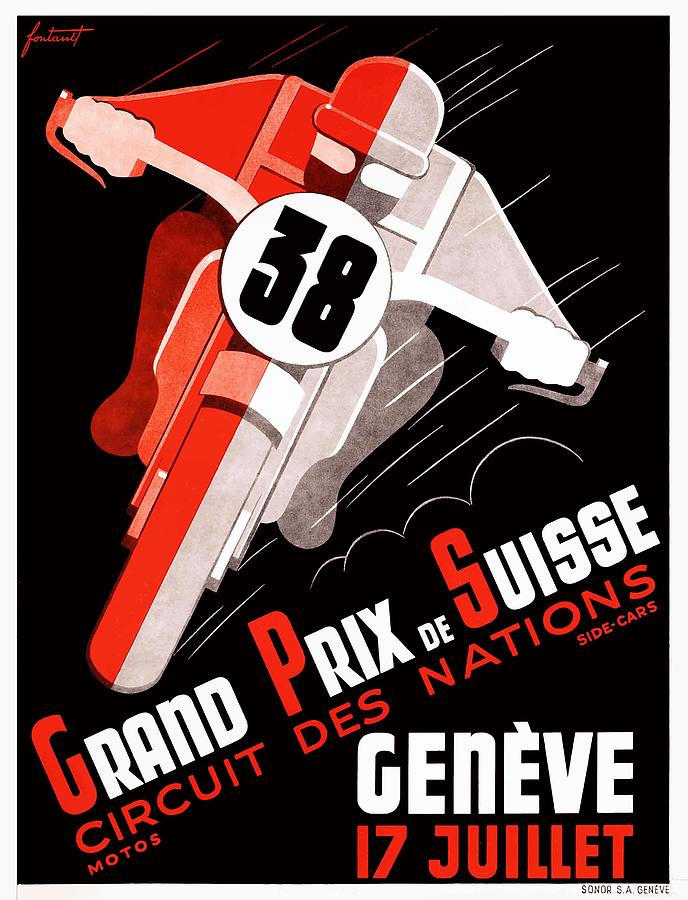This is a highly stylized and cartoonish color poster for a Grand Prix motorcycle race, prominently featuring the number 38 rider. The overall background of the poster is black, while the central image showcases a front-facing motorcycle rider whose left side is vividly illustrated in red and his right side in gray. The rider, complete with helmet and goggles, is mirrored in color on his bike, also characterized by these striking red, gray, and white hues. Below the dynamic image, slanted text in red and white announces the "Grand Prix de Suisse Circuit Donations," emphasizing the event this week. Additional details at the bottom right indicate the location and date: "Genevieve, 17th of July." The dominant colors of red, gray, and black create a bold, eye-catching visual that highlights the excitement and prestige of the race.